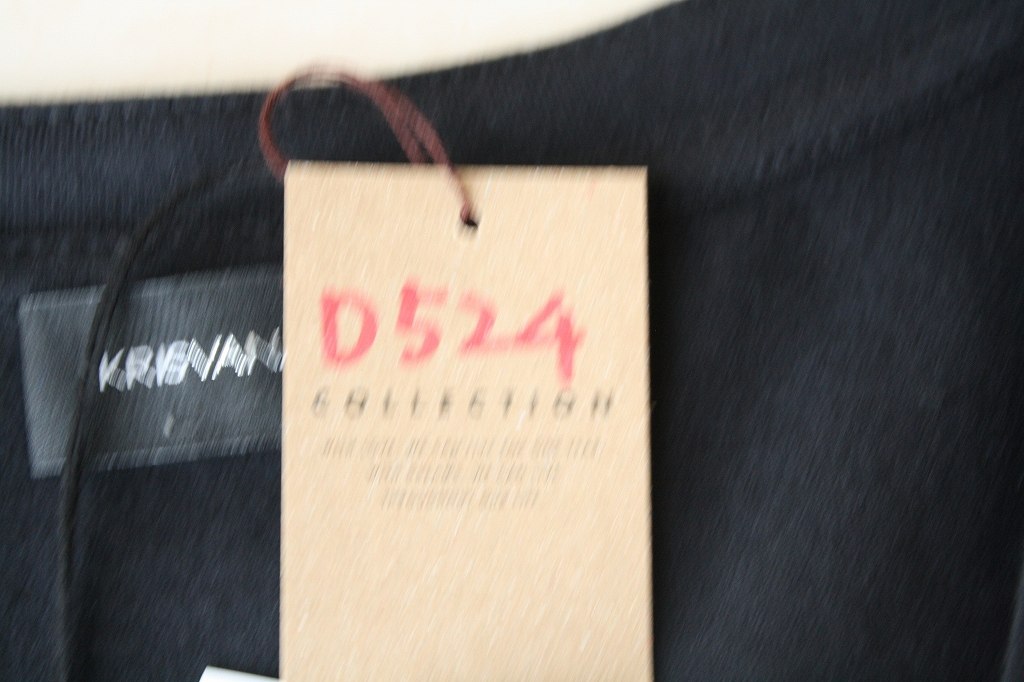This image depicts an extremely blurry, dark-colored piece of clothing, possibly black, featuring a visible collar and multiple tags. On the left side of the garment, a gray sewn-in tag can be observed, albeit fuzzily, with the name "KRIS VAN" inscribed in white. Adjacent to this is a light beige rectangular paper tag attached by a brown string. This tag prominently displays "D524" in red, graffiti-like font, with the word "collection" written underneath in black. Below this, there are three illegible lines of text due to the blurriness. Additionally, a mysterious black strand appears on the left side of the image, but its purpose remains unclear.